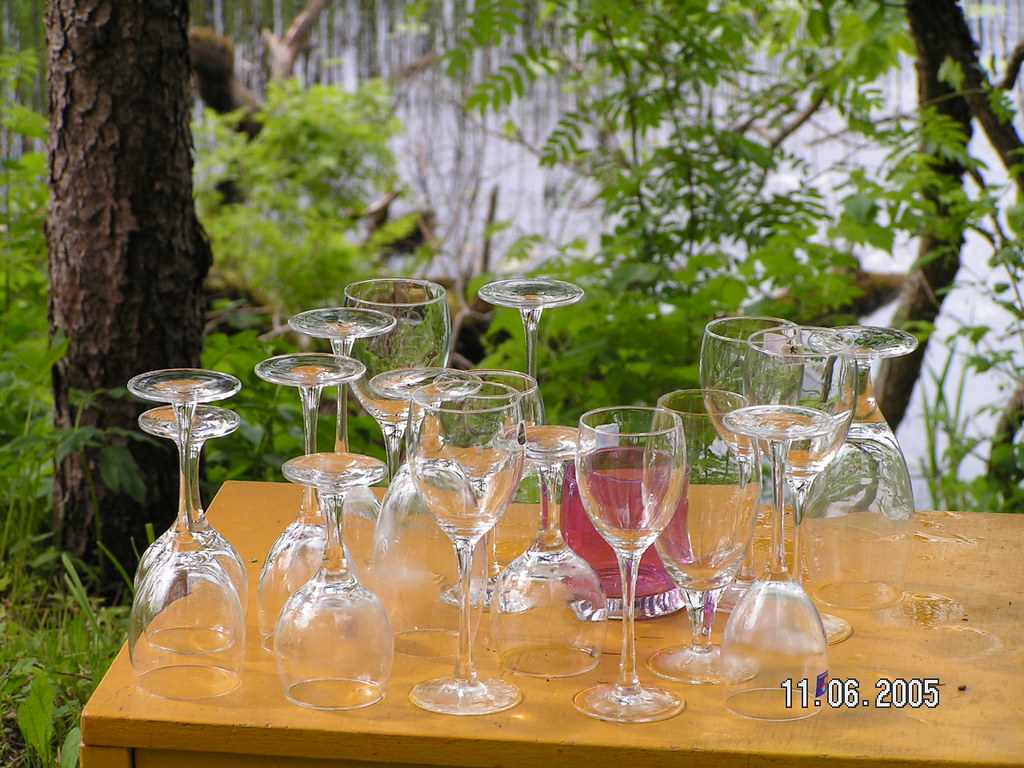This photograph, taken on November 6, 2005, depicts a collection of approximately 12 to 15 glasses meticulously arranged on a medium brown wooden cabinet, set outdoors amid a serene backdrop of trees and shimmering water, suggesting a lakeside or riverside location. The glasses, primarily assorted wine glasses, are placed in a varied but organized manner with both upside-down and right-side-up orientations, hinting at a recent gathering, perhaps a backyard garden wedding reception. From left to right, the arrangement includes two upside-down wine glasses of differing heights, followed by the shortest upside-down wine glass which is mirrored by another further back in the image. There are two slightly taller upside-down wine glasses behind them, and a lone right-side-up wine glass in the rear. To its right, a trio of glasses (two upside down and one right side up) flank another upside-down short wine glass. A distinctive red rocks glass filled with pink liquid stands at the back, anchoring the arrangement. The remainder of the glasses, aligned to the right of the red glass, alternates between right-side-up and upside-down positions. The photograph's focus on the glassware contrasts with the blurred background, balancing the scene aesthetically and drawing attention to the delicate beauty of the arrangement.